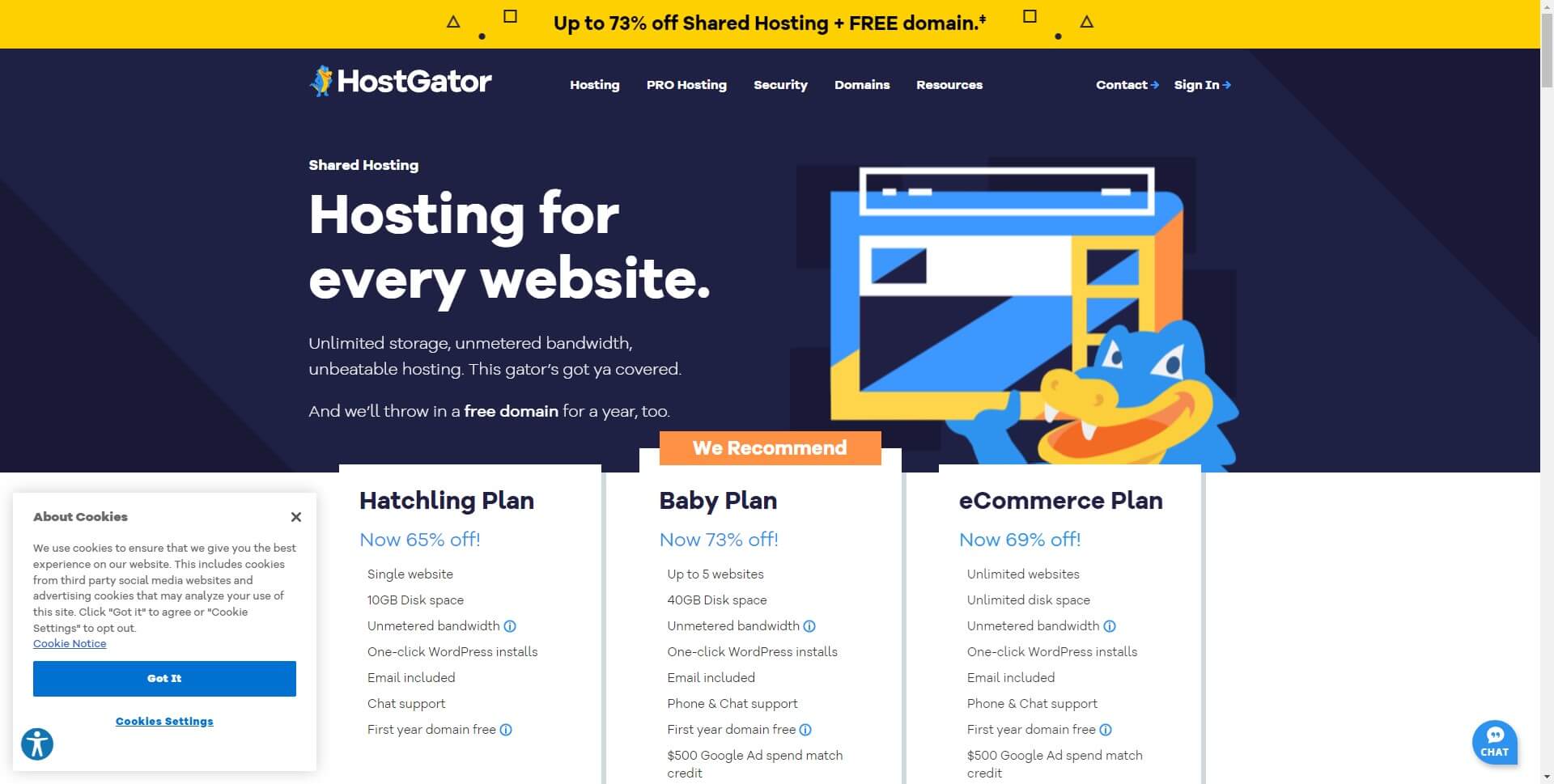The screenshot captures the homepage of HostGator, a renowned web hosting service provider. At the top of the page, a prominent yellowish banner announces a special offer: "Up to 73% Off Shared Hosting Plus Free Domain." This promotion is particularly enticing for those looking to host WordPress sites or any other type of website. 

The main section of the page features the HostGator logo, a cheerful alligator, accompanied by the company name in bold white text against a dark blue background. Below this, a horizontal navigation menu offers various options: "Hosting," "Pro Hosting," "Security," "Domains," "Resources," with additional links for "Contact" and "Sign In," each accompanied by an arrow icon.

Further down, a headline reads: "Shared Hosting for Every Website," highlighting key features such as unlimited storage, unmetered bandwidth, and unbeatable hosting reliability. The text emphasizes HostGator's commitment to providing excellent service with the assurance that "the Gator’s got you covered." A special note mentions an included free domain for the first year or two, adding further value.

At the bottom of the screen, the alligator mascot proudly displays different hosting plans available: the Hatchling Plan, Baby Plan, and E-Commerce Plan, catering to a variety of user needs. The overall layout is clean and inviting, underscoring HostGator's user-friendly approach.